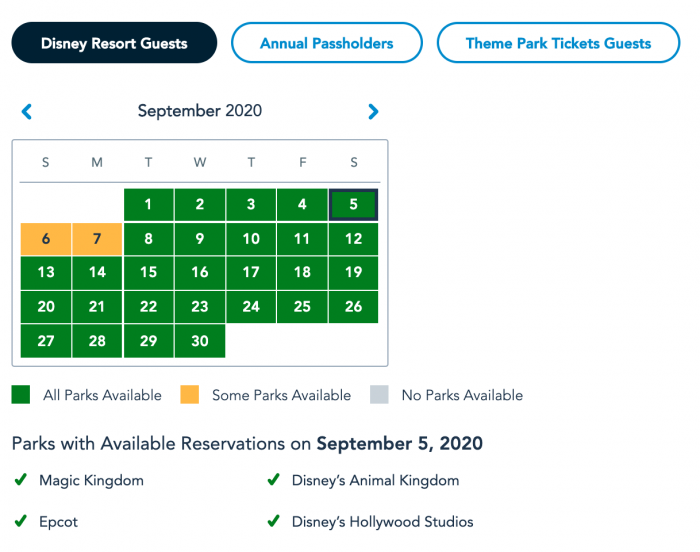The image depicts a travel or reservation website interface for booking Disney Resort experiences. The background is predominantly white. At the top, there are three circular tabs: "Disney Resort Guest," which is highlighted in dark black or blue, "Annual Pass Holders," and "Theme Park Ticket Guest."

Below these tabs, a calendar is displayed. At the top corners of the calendar, arrows allow users to navigate through different months. The current month showcased is "September 2020." The calendar's dates are mostly marked with green square tiles, except for the 6th and 7th, which are in yellow.

A legend below the calendar explains the color coding: green indicates all parks are available, yellow signifies that some parks are available, and gray denotes no park availability. The only dates with restricted park availability are Sunday the 6th and Monday the 7th.

At the bottom of the image, there are checkmarks beside icons for Animal Kingdom, Magic Kingdom, Epcot, and Hollywood Studios, indicating these parks are options within the reservation system.